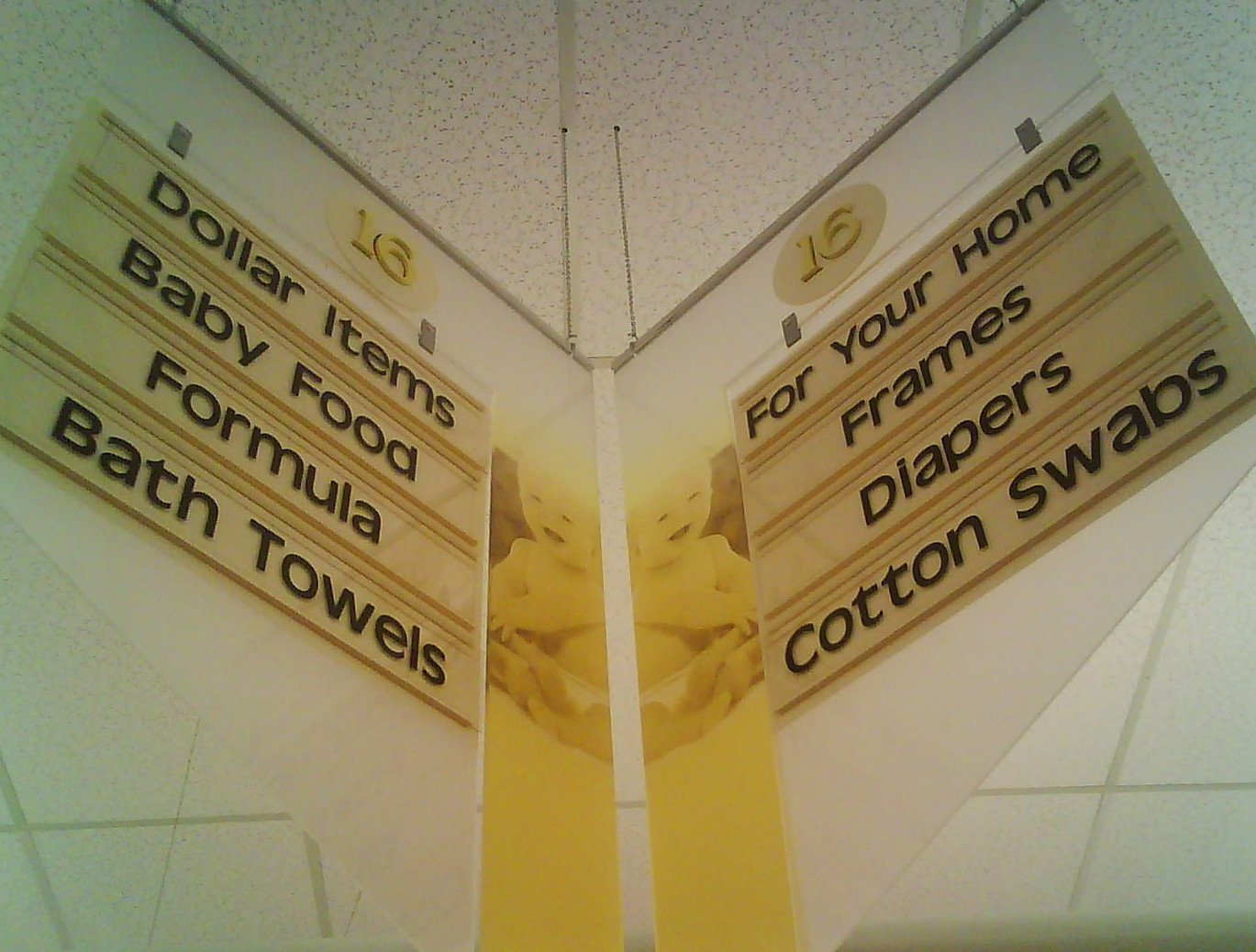This color photograph, taken inside a store or a pharmacy, features a prominent overhead aisle sign. The sign is divided into two sections, left and right, both labeled for aisle 16. The background is a stark white, with a popcorn-textured ceiling adding detail to the upper frame.

Long plastic strips, four on each side, create diagonal lines that converge towards the bottom center of the image, drawing attention to the sign's content. The left side of the sign, marked by a yellow number 16, lists "Dollar Items," "Baby Food," "Formula," and "Bath Towels" in black text. Adjacent to each portion is a gradient yellow photograph of a baby, enhancing the baby-related items listed.

On the right side, also under a yellow number 16, the sign reads "For Your Home," "Frames," "Diapers," and "Cotton Swabs," again in black text. Both parts of the sign are securely suspended from the ceiling by metal chains, ensuring they remain visible to shoppers navigating the aisle. The detailed arrangement and vivid categorization make it easy for customers to locate the items they need.